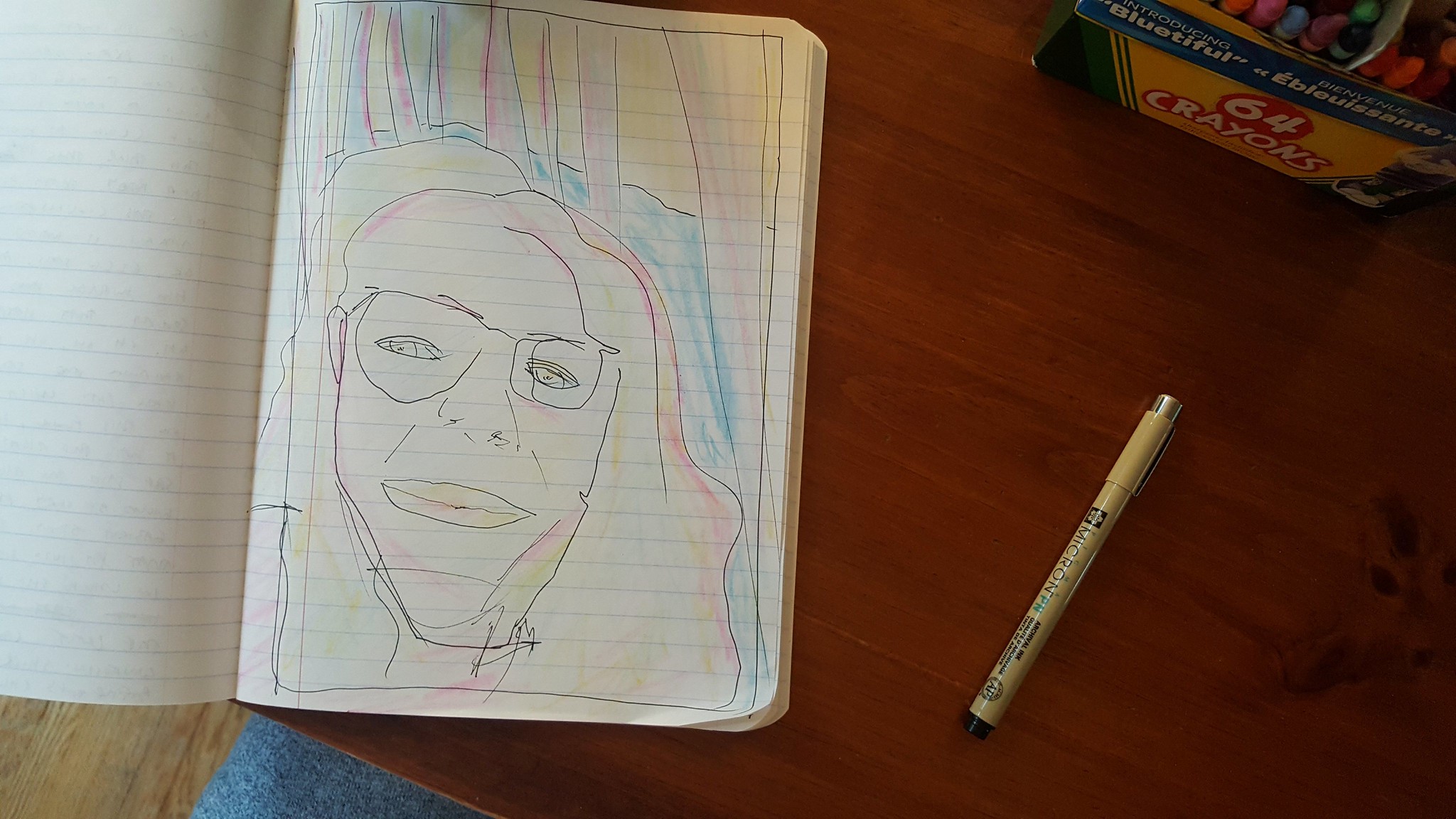The photo captures a sketch in an open lined notebook, placed on a brown wooden table with visible grain. To the right of the notebook lies a yellow Micron PN pen, and in the upper right-hand corner, there’s a yellow box of 64 crayons, showcasing a few colors like blue, purple, and orange. The notebook, positioned slightly to the left in the frame, features a crude drawing of a person's face on the right-hand page. The sketch depicts a person with glasses, large lips, a prominent nose, and some wrinkles on the cheek. The person’s hair is detailed with yellow and pink crayon, and there’s a hint of blue coloring in the background. The face, looking slightly to the left, appears to be a novice effort, likely the artist's first attempt.